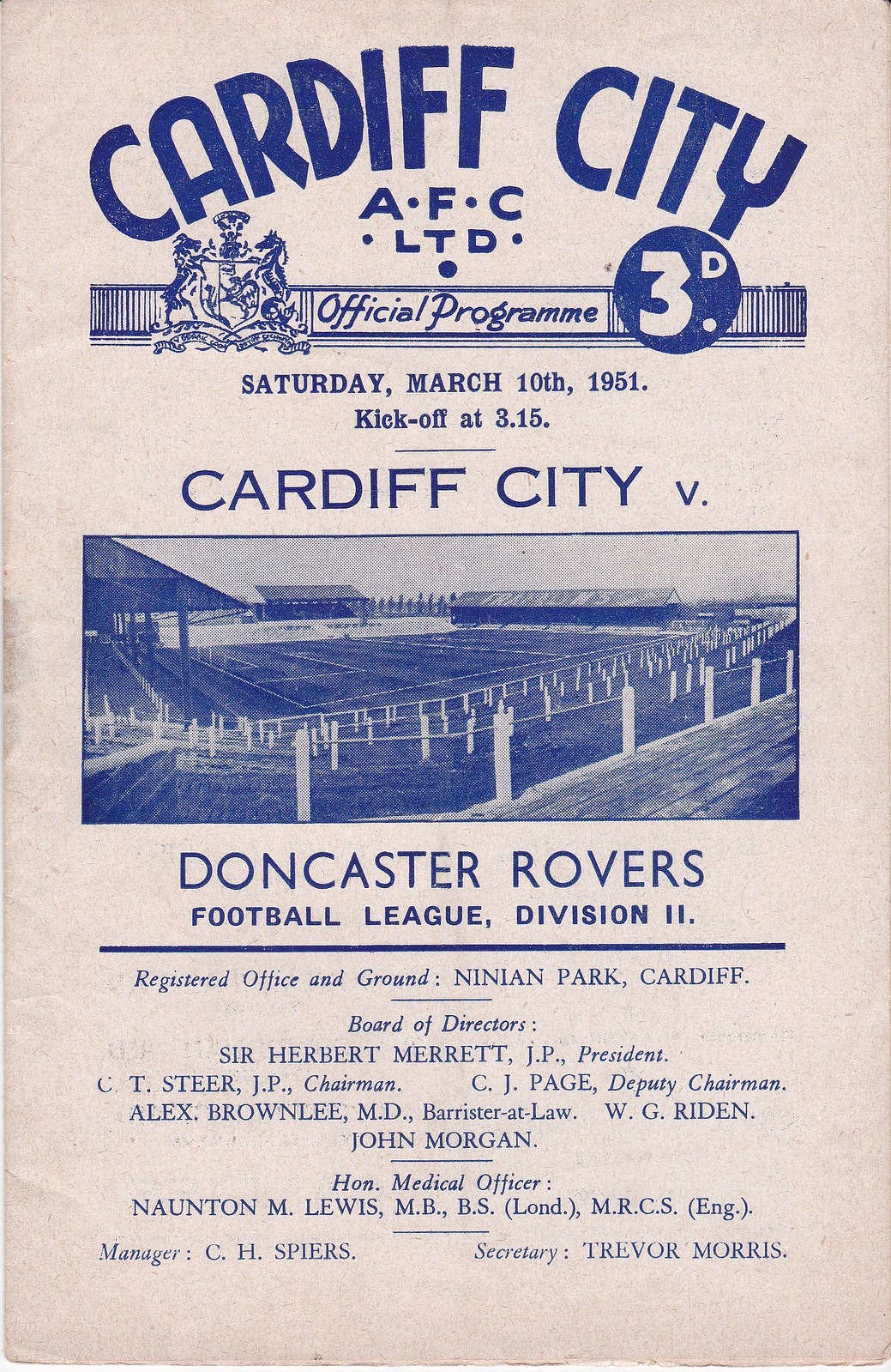The image showcases the front cover of a vintage football program for a match held on Saturday, March 10, 1951, with a kickoff time of 3:15 PM. The cover is vertically oriented and has a light pink to beige background with dark blue text and graphics. At the top, "Cardiff City AFC LTD" is emblazoned in thick, boxy typeface, followed by the phrase "Official Programme" in smaller lettering, adhering to the English spelling. Adjacent to this is a dark blue circle with "3D." The date and time details are printed below in all caps: "SATURDAY, MARCH 10, 1951 KICKOFF AT 3.15."

Underneath, "CARDIFF CITY" in thin, boxy letters announces the home team, followed by a stylized representation of the playing field from the stands. The teams are contrasted by "VERSE" and "DONCASTER ROVERS" in similar thin, boxy typeface. Below this is the notation "FOOTBALL LEAGUE DIVISION 2."

Further down, the program lists key personnel including:

- Sir Herbert Merritt, President
- C.T. Steer, Chairman
- C.J. Page, Deputy Chairman
- Alex Brownlee, Barrister at Law
- W.G. Rydin
- John Morgan, Honorary Medical Officer 
- Naunton M. Lewis, Manager
- C.H. Spears, Secretary 
- Trevor Morris

The cover is marked by some wrinkling, particularly on the left side, and the overall design reflects its age, with a cream-colored, slightly yellowed background and blue-tinted, monochromatic imagery.